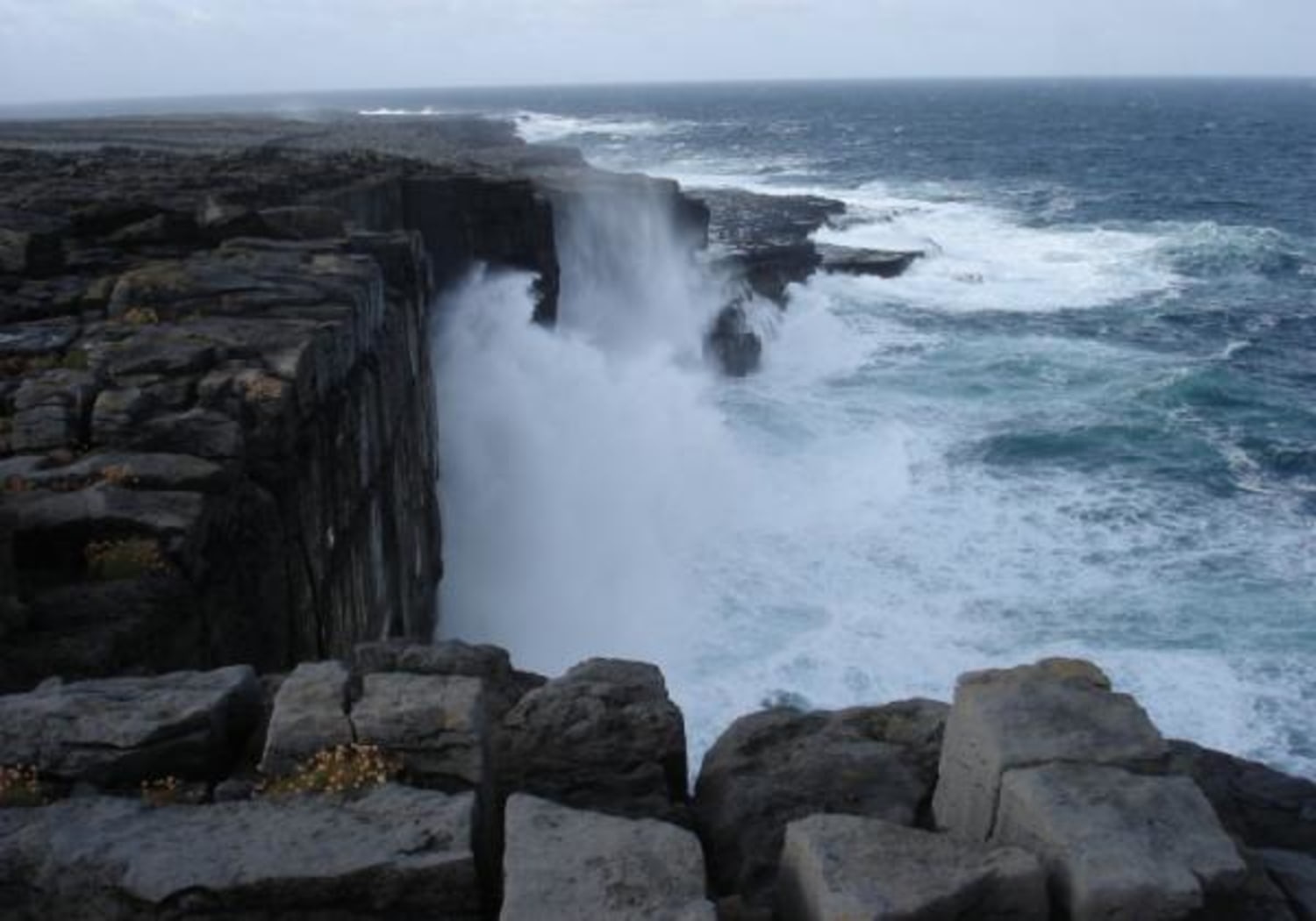The photograph is a horizontal rectangular image capturing an impressive cliffside scene where the land meets the ocean. On the left side of the image, a steep cliff face dominates, showing a dramatic drop-off. To the right, the ocean stretches out, with waves relentlessly crashing into the cliff, sending white spray and foam skyward. The water is a mix of dark blues and greens, suggesting a turbulent yet clear sea. The waves vary in size, with some forming dark, looming shapes and others breaking into smaller, frothy surges against the rugged rocks. In the background, more flat areas of the ocean are visible, fading into the horizon where the sky, slightly overcast with white clouds, meets the sea. The scene is accented by a patch of greenery that clings to the top of one of the rocks, adding a touch of life to the rocky seascape. The overall atmosphere of the image is one of raw natural beauty and power, showcasing the relentless force of the ocean against an unyielding stone.